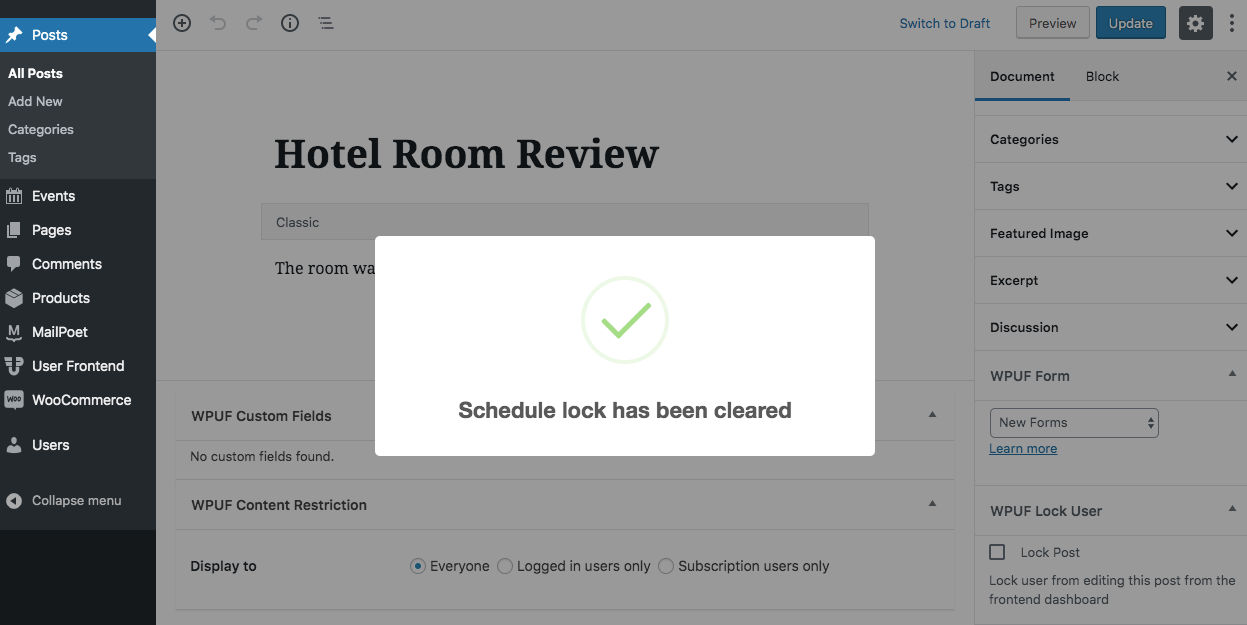**Caption:**

A detailed screenshot of a WordPress blog's control panel, showcasing the user interface and available options. On the left-hand side, a vertical gray menu is present with the top item, "Posts," highlighted in blue. The "Posts" section is expanded to reveal sub-options: All Posts, Add New, Categories, and Tags. Below these are other menu items: Events, Pages, Comments, Products, MailPoet, MailPost, User Front End, WooCommerce, Users, and a button labeled "Collapse Menu."

In the main workspace, a grayed-out interface is overlain by a large white rectangular notification with a green check mark that reads "Schedule Lock has been cleared." The workspace beneath this overlay includes options to Switch to Draft, Preview, and Update the post. A gear icon is positioned at the top-right of this section.

The post under review is titled "Hotel Room Review" with input fields and options detailed below. The primary content editor is set to "Classic" format, with placeholder text indicating "The room was something." Beneath this, sections for WPUF (WP User Frontend) custom fields and content description are noted, though no custom fields are found.

A secondary menu on the right-hand side provides further options categorized under Document, Block, Categories, Tags, Featured Image, Excerpt, Discussion, WPUF Form, New Forms, and WPUF Lock User. Additionally, there is an unchecked box labeled "Lock Post" with the instruction to lock the user from editing this post from the front-end dashboard.